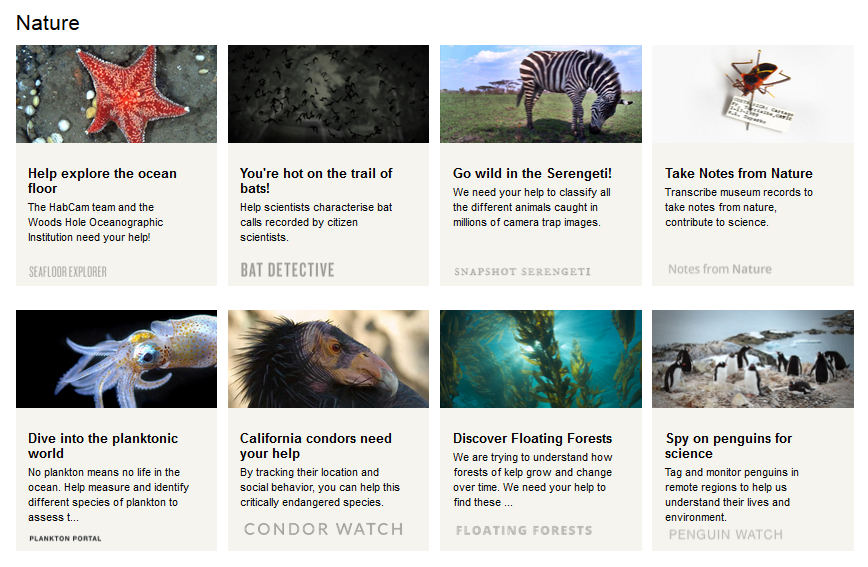Here is a more detailed and cleaned-up caption for the described images:

"Embark on a visual journey through diverse natural environments. The first image invites you to 'Help Explore the Ocean Floor,' featuring a vibrant starfish set against the seabed. The second image captures bats in mid-flight against a black and white sky, accompanied by the phrase 'You’re Hot on the Trail of Bats.' Next, a serene scene shows a zebra grazing on grass, labeled 'Go Wild in the Serengeti.' Following this is a detailed image of a pinned insect with an attached note, urging viewers to 'Take Notes from Nature.' A subsequent image depicts tiny plankton in their aquatic habitat and encourages us to 'Dive into the Planktonic World.' The majestic California condor is next, highlighted with the statement 'California Condors Need Your Help.' An underwater vista of vibrant blue seaweed bathed in sunlight follows, urging viewers to 'Discover Floating Forests.' Finally, the last image features a group of penguins on rocks and in the water, with the call to 'Spy on the Penguins for Science.' Each image vividly portrays the beauty and diversity of our natural world, encouraging exploration and conservation."